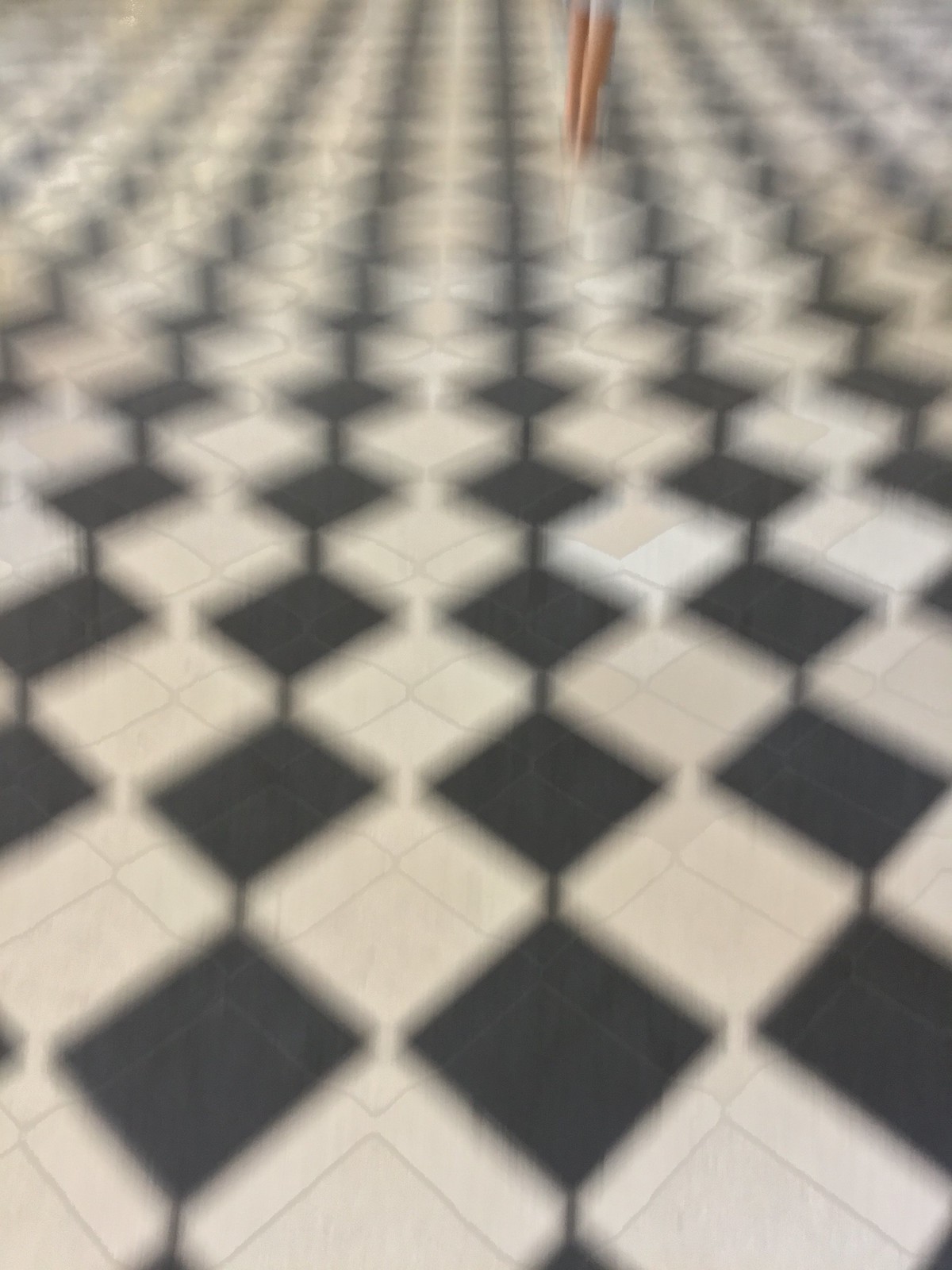The image depicts a somewhat blurry photograph of a floor, likely a linoleum or vinyl tile surface. The clarity of the image improves from the bottom towards the center but becomes increasingly blurred towards the top. The floor features a pattern of black square tiles that are rotated so that their corners point vertically and horizontally, creating a diamond-like appearance. Surrounding these black tiles are white tiles, providing a stark contrast that accentuates the diamond pattern. The white tiles have a textured finish, adding a subtle depth to the overall design of the floor. Despite the blurriness at the top, the distinct pattern and texture of the floor remain recognizable.